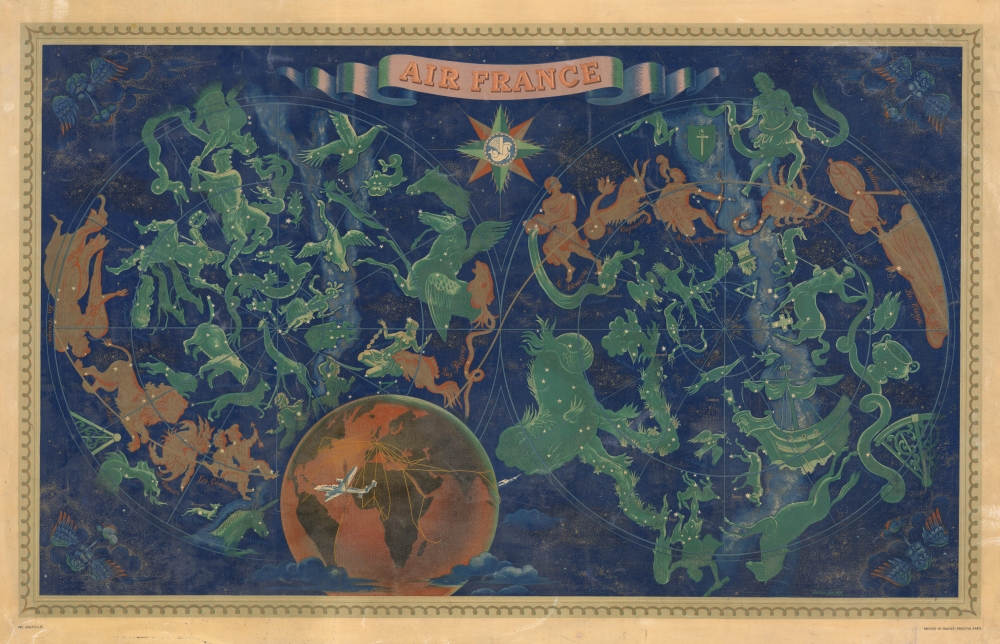The image depicts a detailed painting set against a predominantly navy blue background. At the top of the rectangular frame, a banner reads "Air France," beneath which there is a compass-like star. The border of the painting is a mix of coral and brown with intricate dark brown curly patterns, giving it a textured frame-like appearance. Notably, the image contains two main globes. The bottom left of the picture features a red, brown, and bronze globe showing an airliner between Africa and South America. In addition, there is another globe depicted in coral and moss green colors, with white and gray airplanes above it. Surrounding these globes are various green, brown, and orange shapes resembling humans, animals, birds, and majestic figures, contributing to a rich tapestry that merges map-like details with artistic elements.